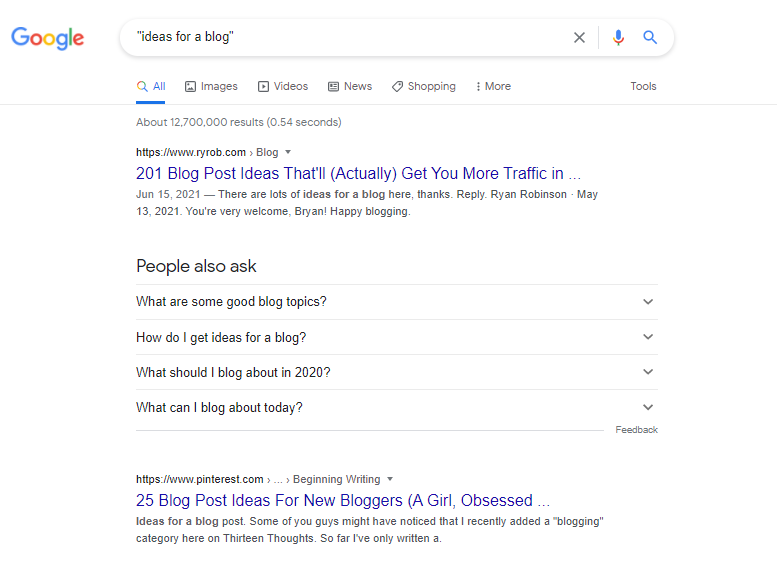The image displays a Google search results page with a white background and predominantly black text. At the top, next to the Google logo, the search box contains the query in quotations: "ideas for a blog." The search results are shown under the "All" category, rather than images, videos, news, or shopping. 

The first search result is a blog post from ryrob.com, titled "201 Blog Post Ideas That'll (Actually) Get You More Traffic." This article is prominently displayed at the top of the search results. Below that, there's a section labeled "People Also Ask," featuring related questions that other users have searched for, including:

- What are some good blog topics?
- How do I get ideas for a blog?
- What should I blog about in 2020?
- What can I blog about today?

These questions can be expanded to view more specific answers. Following the "People Also Ask" section, the second search result is from Pinterest, titled "25 Blog Post Ideas for New Bloggers."